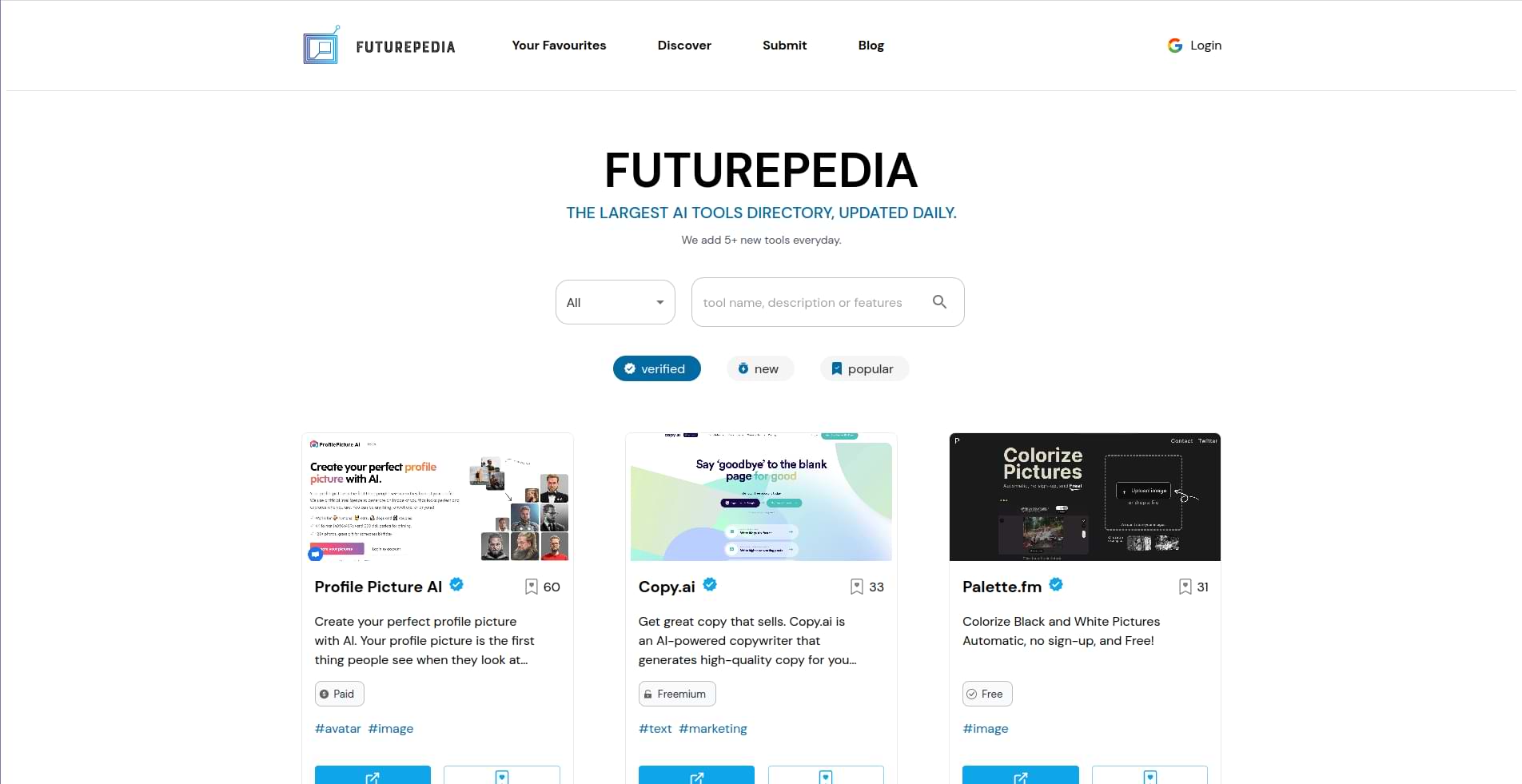This is an image of the Futurpedia website interface. At the top of the page, various tabs are visible, including "Your Favorites," "Discover," "Submit," and "Blog." On the side, there's a "Login" option. Below the main website header, the bold title "Futurpedia" is prominently displayed with the tagline "The largest AI tools directory updated daily" underneath it.

A search functionality is available, starting with a dropdown box labeled "All" next to a large search bar where users can input tool names, descriptions, features, and other keywords. Beneath this search section, three buttons are present: "Verified," "New," and "Popular." The "Verified" button is highlighted in blue, whereas the other two are in gray.

Under these buttons, three highlighted tools are showcased in separate boxes. The first tool, "Profile Picture AI," is described as a tool for creating profile pictures. The second, "Copy.ai," is identified as a tool for copywriting. Lastly, "Palette.fm" is presented as a service for colorizing black-and-white photos. Each tool listing includes a corresponding icon or image, providing a visual representation of the tool's function.